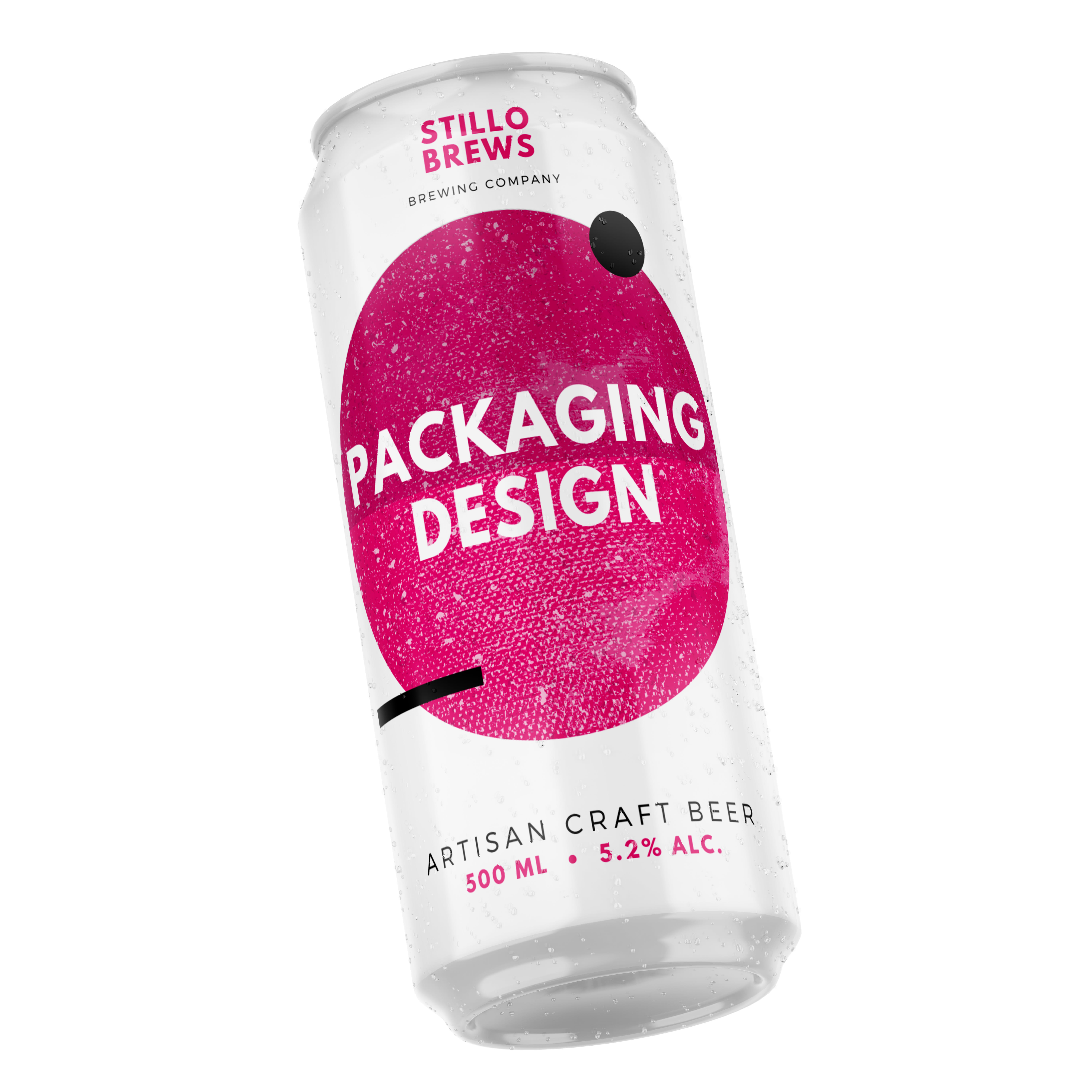This is a professionally staged and full-color photograph of a tall, white, and silver beer can against a solid white background with no border. The can is adorned with condensation droplets, giving it a refreshing look. At the top of the can, in dark pink, all-caps letters, it says "STILLO BREWS." Directly below that, in black, all-caps letters, it reads "BREWING COMPANY." A large dark pink, speckled oval dominates the can's front, displaying the phrase "PACKAGING DESIGN" in white, all-caps letters. This oval also features a white horizontal line, partially inside and outside the oval. There is a black circle on the upper right of the oval and a black vertical rectangle near the bottom. At the very bottom of the can, in black, all-caps letters, it says "ARTISAN CRAFT BEER," followed by "500 ML" and "5.2% ALC" in dark pink. The metallic elements and overall design suggest this is a high-end, craft beer brand, possibly showcased for promotional purposes.